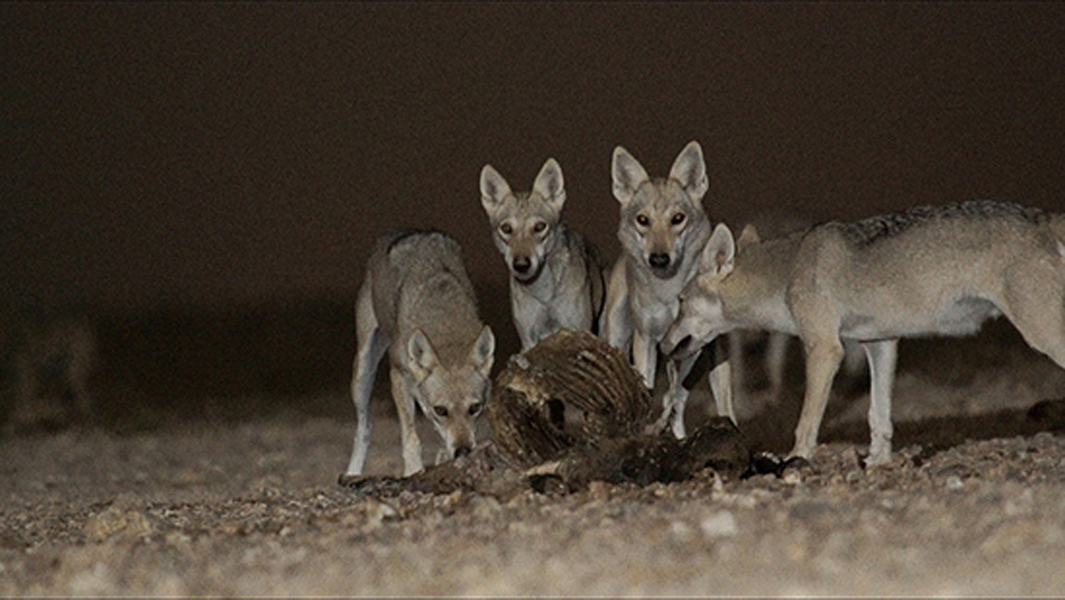The photograph depicts a nighttime scene featuring four grey wolves gathered around a long-dead animal carcass, predominantly consisting of exposed rib bones. The ground appears gravelly and flat, and the overall atmosphere is dim with a grey texture. Two of the wolves appear to be trying to dig into the carcass, while the other two direct their gaze towards the photographer. Despite the gory nature of the scene, the wolves maintain a dog-like appearance, evoking a mix of danger and intrigue.